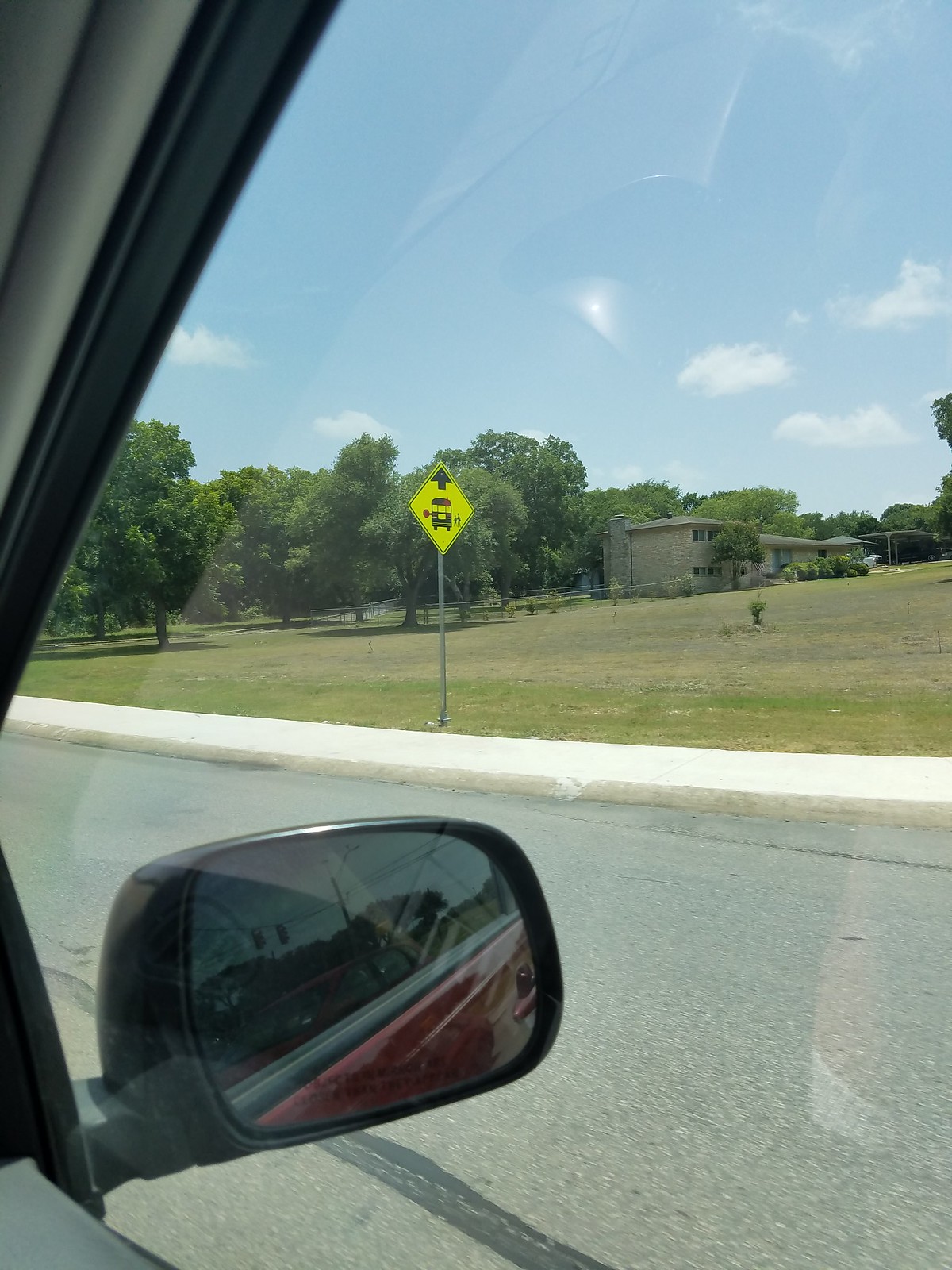The image shows a scenic view from the passenger side window of a red car, revealing both the side mirror and its reflection. The car is driving on a street that features a concrete sidewalk bordered by a lush, green grassy area with patches of light brown. Prominently displayed in the center of the image is a diamond-shaped yellow sign on a gray pole, which features a black upward-pointing arrow above an illustration of a school bus with its red stop sign extended, indicating a school bus stop ahead. The backdrop includes a number of tall, verdant trees located towards the left side, alongside a light brown brick house with a chimney, and what looks like a carport near the right. The sky is clear with a few clouds, adding to the daytime ambiance.